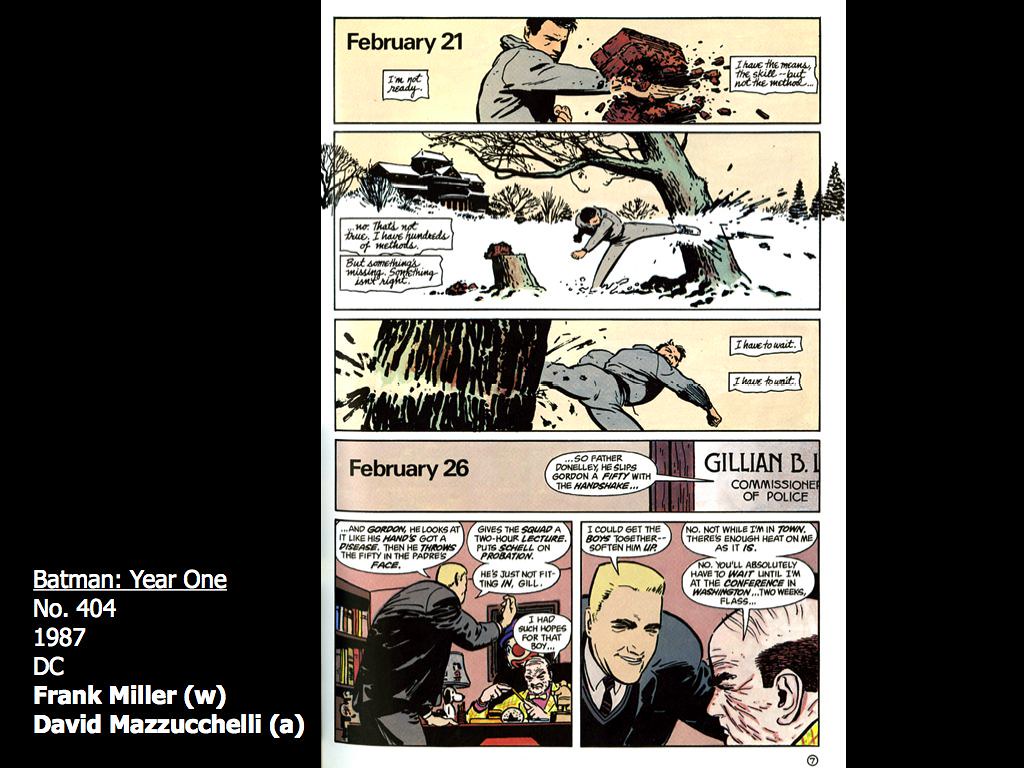This color illustration, set against a large black background, features a classic cartoon clipping. The title, "Batman: Year One, Issue #404 (1987)," is written in white in the lower right corner of the black backdrop, and credits Frank Miller (w) and David Mazzucchelli (a).

The cartoon segments are laid out in two separate panels on the black background. The first panel, dated February 21st, is divided into three horizontal strips, each depicting sequential scenes. The second panel, dated February 26th, is organized with one horizontal strip at the top and two square frames side by side beneath it.

Overall, the image captures a pivotal moment from the iconic Batman series, brought to life by the distinguished collaboration of Miller and Mazzucchelli, showcasing their renowned storytelling and artistic skills.